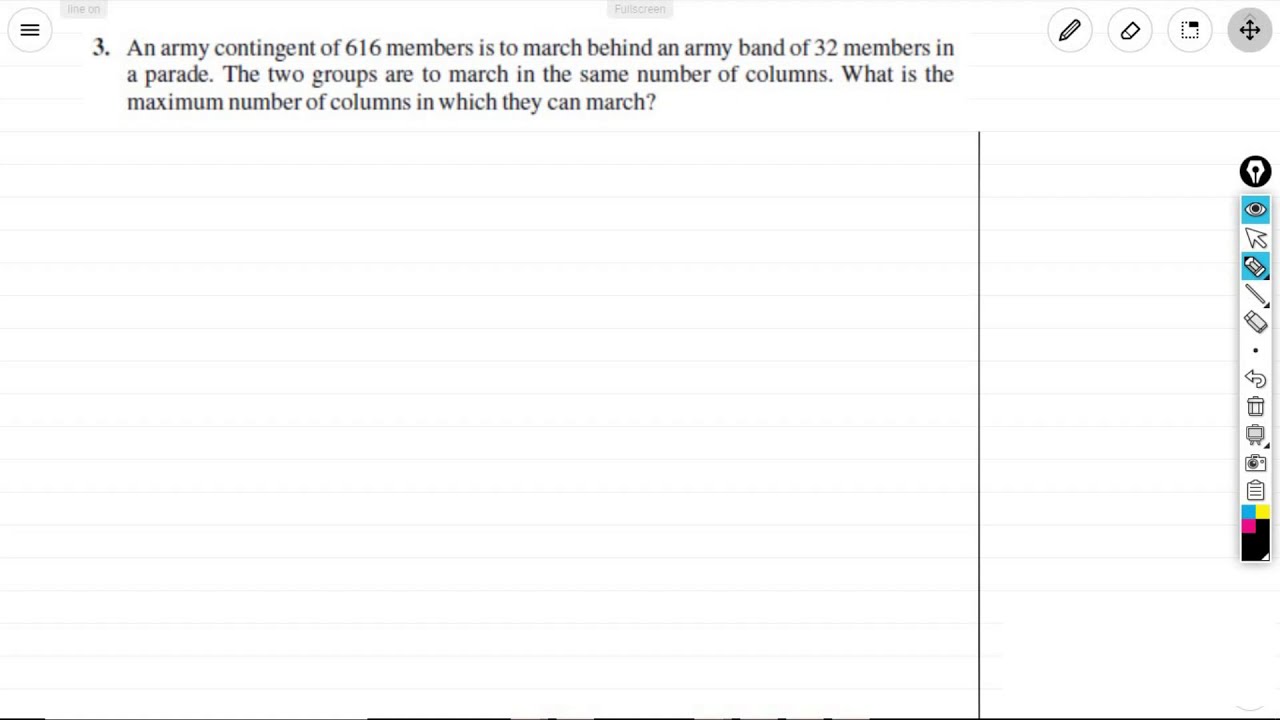The image is a full-screen screenshot of a computer program that appears to be an editing or writing software, possibly used for online learning or completing assignments. The interface includes various tool icons, such as a pencil, an eye, an arrow, an eraser, a waste bin, a camera, and a clipboard, along with simplified color options. In the top right corner, there are controls for zooming, scrolling, erasing, clipping, cropping, and writing on the document. The visible text on the screen is a math problem labeled as "number three" which states: "An army contingent of 616 members is to march behind an army band of 32 members in a parade. The two groups are to march in the same number of columns. What is the maximum number of columns in which they can march?" The rest of the document is blank, indicating that it might be awaiting input or a solution from the user.